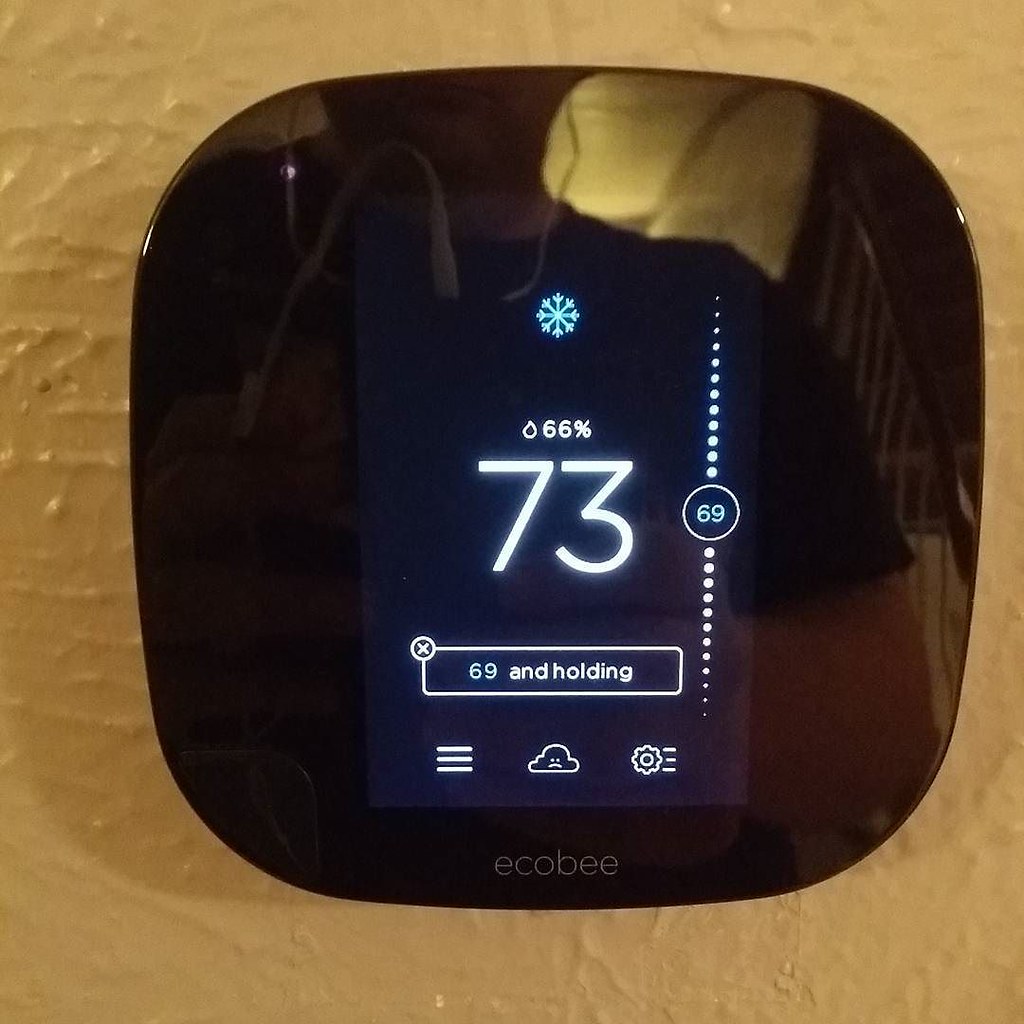The image showcases a close-up view of a sleek, black, shiny plastic temperature and humidity device from the Ecobee brand, mounted on a brown stucco-type wall. The device prominently displays the temperature and humidity levels in large, white numerals with accompanying white dots and circles, supplemented with pale blue numerals and symbols for additional clarity.

The main temperature reading, positioned at the center in very large numbers, is 73°F. Just above this, in smaller font, a raindrop icon indicates the humidity level at 66%. At the very top center of the display, a pale blue snowflake icon is visible. 

Directly below the 73°F reading, a rectangular box features the number 69 in pale blue inside a white outline, with the word "holding" in white lettering next to it. Beneath this box, three dashes arranged in a vertical column can be seen, with a cloud bearing a frowny face icon in the middle.

To the right of the cloud icon, there is a settings gear icon accompanied by three horizontal dashes. Running parallel along the right side, from the snowflake at the top to just below the rectangular box with the number 69, there is a vertical scale with circles that increase in diameter from top to bottom. The largest circle, located at the center right, is filled in white, encasing the number 69 in pale blue.

The overall design of the display on the Ecobee device is not only functional but also aesthetically integrated to provide an easy-to-read and detailed overview of both indoor temperature and humidity conditions.